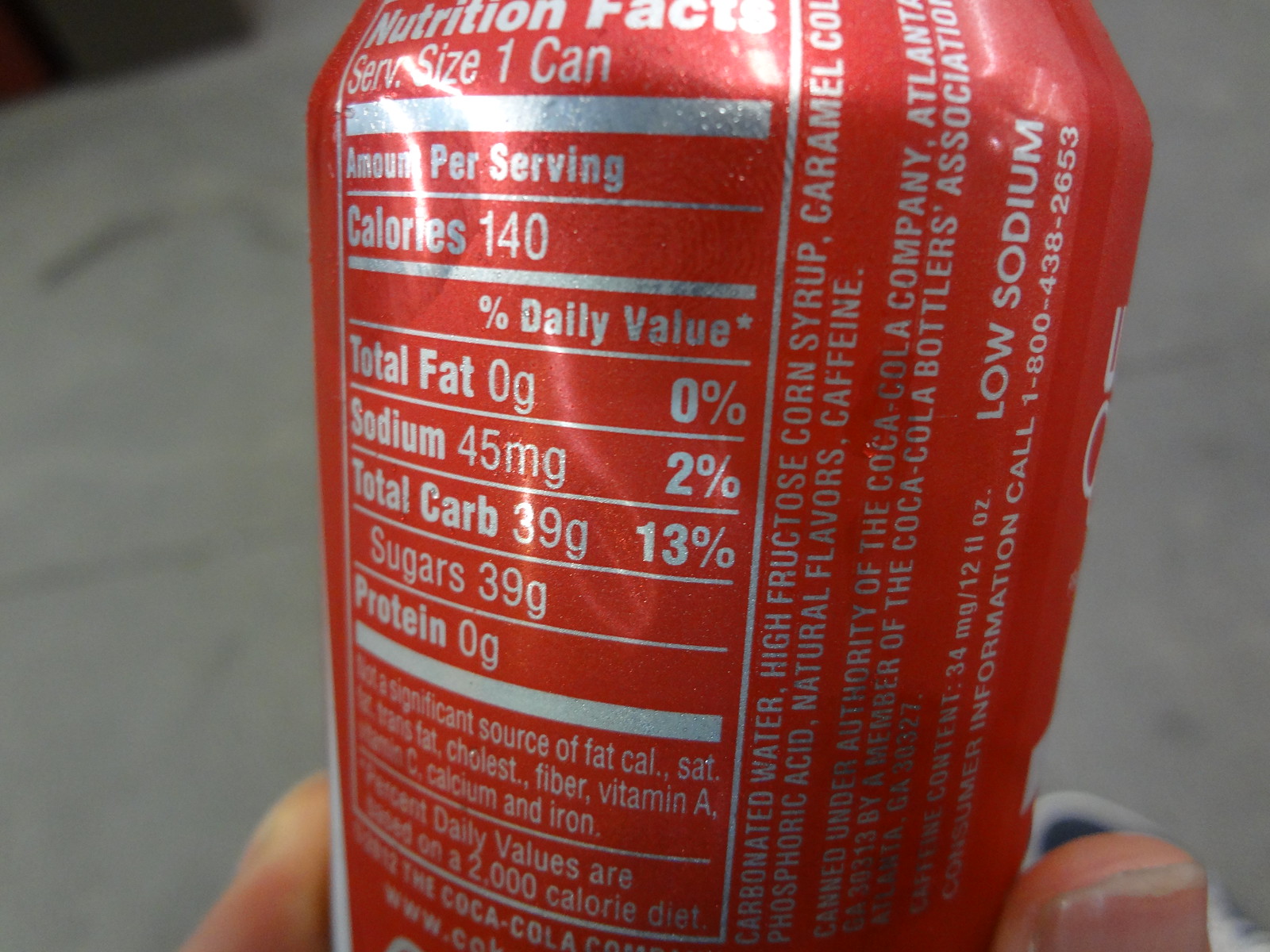This detailed image features a close-up of a red Coca-Cola can held by a person's partially visible thumb and finger against a gray background. The focal point is the can, showcasing its Nutrition Facts label, which reads: serving size 1 can (140 calories, 0 grams total fat, 45 milligrams sodium, 39 grams total carbohydrates, 39 grams sugars, 0 grams protein). Also detailed in the ingredients section are carbonated water, high fructose corn syrup, caramel color, phosphoric acid, natural flavors, and caffeine. The text further notes a low sodium content. The photo's composition, slightly blurred at the edges, emphasizes the can’s label and the hand holding it, capturing every intricate detail of the nutritional information and the can's iconic red color.